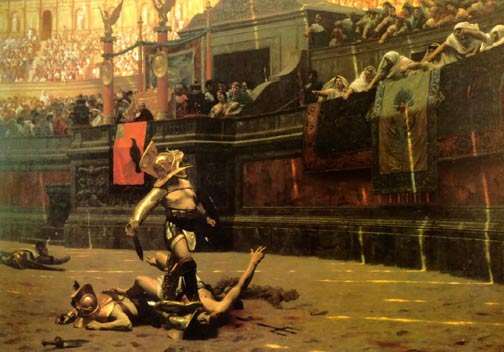In this detailed painting, reminiscent of a Roman-era gladiatorial arena, the dramatic scene unfolds partially on the sandy, light-brown floor of the Colosseum. At the forefront, a muscular gladiator, bare-chested save for metal armor on his right arm and a formidable gold helmet covering his entire head, stands victoriously. His short sword is gripped tightly in his right hand, and he gazes slightly to the side, up towards the roaring crowd. Dominating the composition, his foot rests menacingly on the neck of a fallen foe, a man in similar Roman attire laying lifeless on the ground. Another defeated gladiator is sprawled face-down nearby, also clad in matching armor and helmet. Blood from their bodies seeps into the ground, underscoring the brutal combat.

Encircling the battleground is a red and black concrete wall, above which throngs of spectators in white togas lean in, their faces alive with excitement and cheers. The stands are packed, ascending in tiers that culminate in banners and flags fluttering against the walls. One notable banner, adorned with an orange crow, sways in the fray. Among the crowd, the emperor’s box stands out, adorned with decorations and sheltering a figure wearing a crown. The infectious energy of the spectators fills the air, capturing the visceral intensity of a gladiator’s fight for survival in this vividly evocative painting.